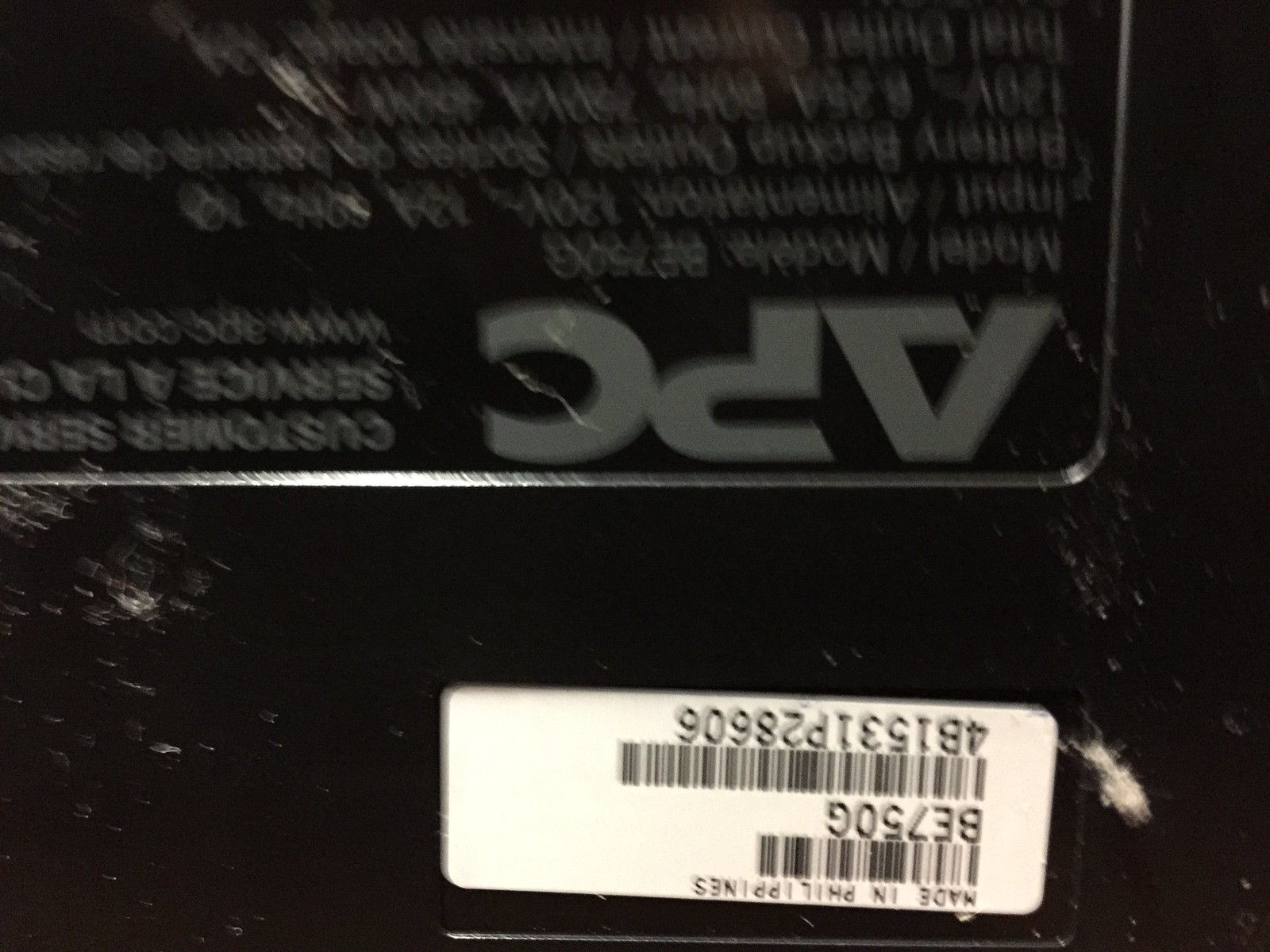The image showcases the backside of an electronic device or household item, photographed with the orientation flipped upside down. Key details include a label in the bottom right corner that reads "Made in the Philippines." This section also features a barcode beneath which the model number "BE750G" is listed alongside a larger barcode. Above this, the identification number "4B1531P28606" is visible. The brand "APC" is displayed prominently above, indicating it belongs to their "Customer Series." Further information includes a service number and a web address leading to www.apc.com. The label provides comprehensive details about the model, voltage, amperage, and battery specifications. The image is set against a black backdrop, with most text in gray or white fonts contrasted against the black background, and the barcodes printed in black on white paper.